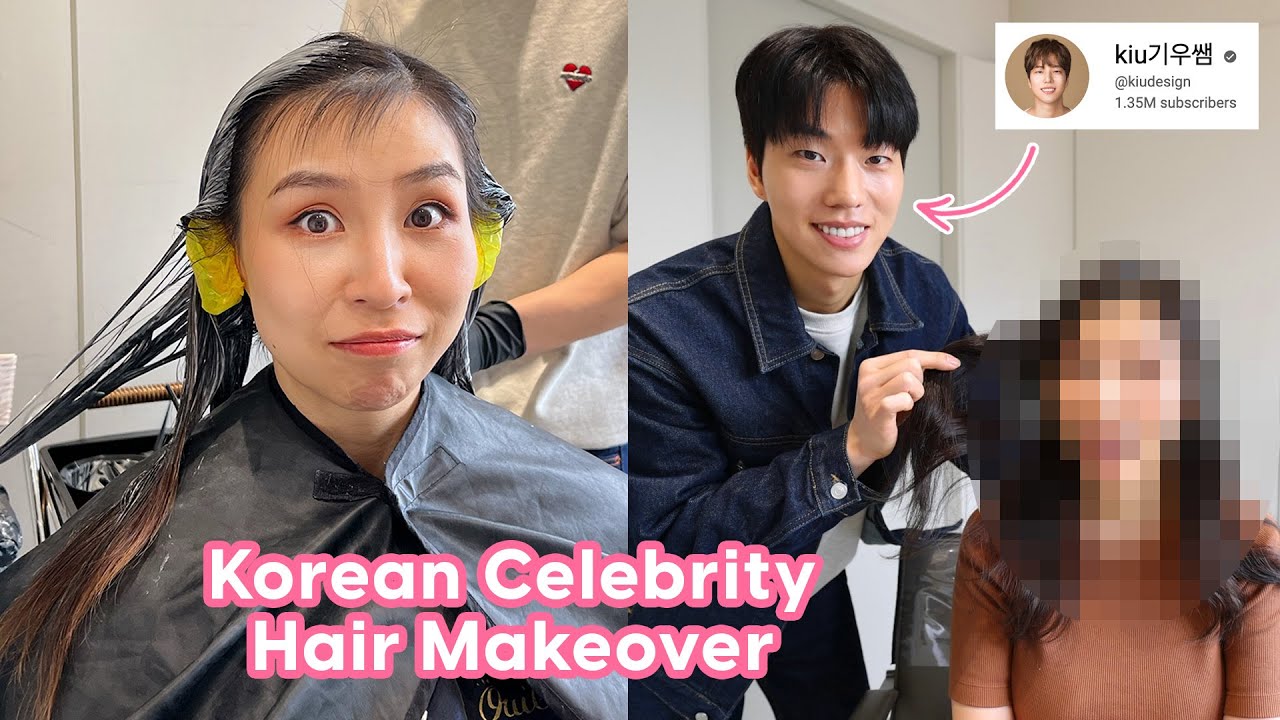The image is a horizontally rectangular, digitally enhanced collage composed of two vertically rectangular, full-color photographs placed side by side. The left photo features a Korean woman in the midst of a hair makeover, with her hair wet and wrapped in yellow plastic to protect her ears, while a man in black gloves, presumably the stylist, works on her hair. She's wearing a black cape to keep her clothes dry. The right photo depicts the same woman post-makeover, though her face is heavily pixelated. A man, identified in the text box in the upper right corner as having 1.35 million subscribers at K-I-U Design, is standing beside her, smiling broadly and holding her hair. An arrow points from this text box to the man, indicating that he is likely the hairstylist. At the bottom left corner is a caption in white text with a pink border that reads, "Korean Celebrity Hair Makeover."